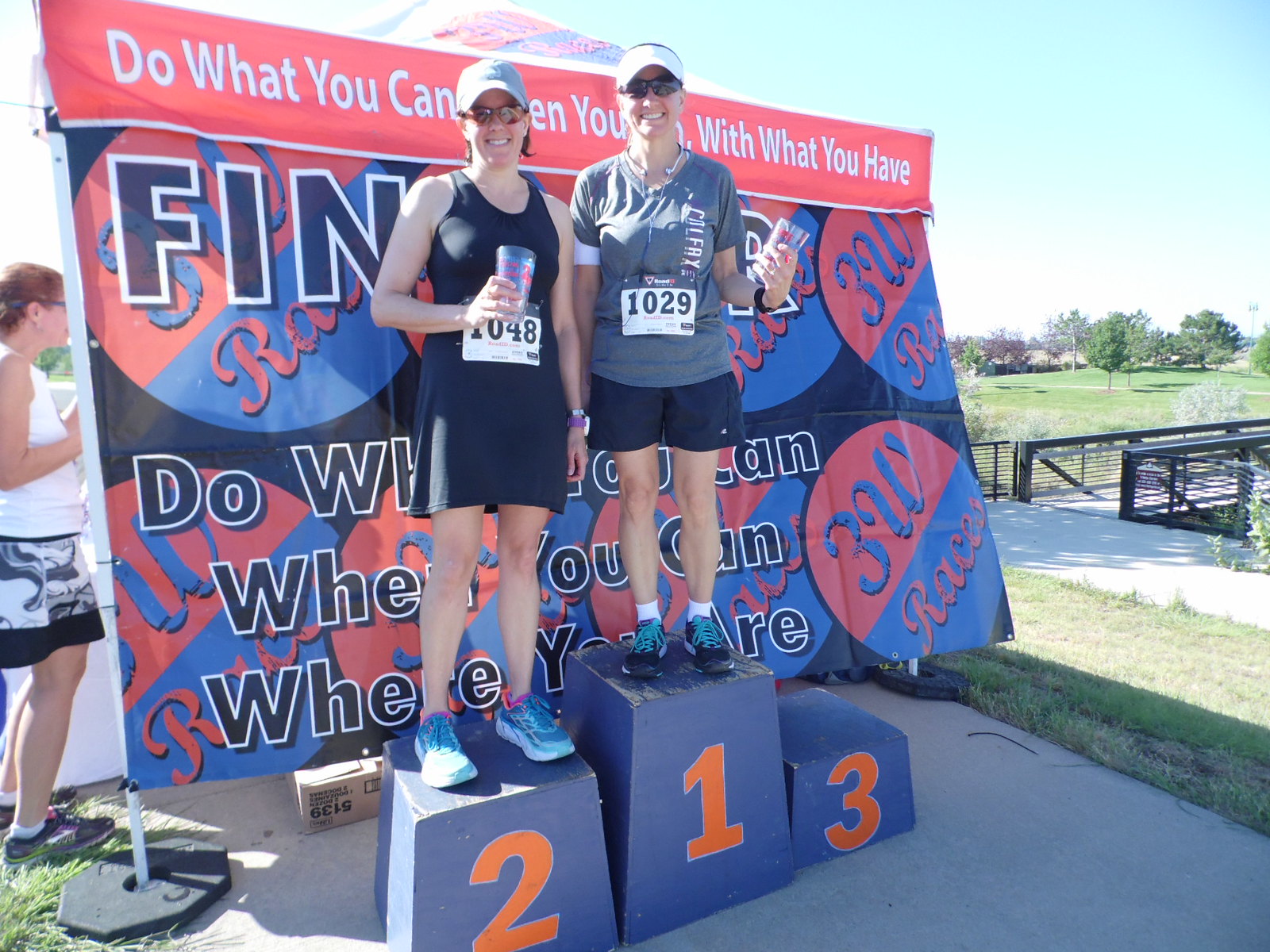The photo captures an outdoor competition award ceremony, centering on a podium with three blocks for places—labeled 1, 2, and 3 from center to left to right. On the highest block, marked number 1, stands a woman wearing a white visor, dark sunglasses, a gray t-shirt, black shorts, white socks, and black shoes with teal shoelaces. She holds a card in front of her labeled "1029" and appears to have short hair and a necklace. To her left on the slightly lower block numbered 2, stands another woman in a white cap, sunglasses, a black tank top, black skirt, and blue shoes, holding a glass in front of her. Her card, partially visible, reads "048". Both women are white and smiling.

Behind them, a large banner displays a partially obstructed motivational message: "Do what you can, even when... with what you have." The banner includes circular symbols with hints of text like "F-I-N," "do," and "W-H-E." The background features a green park with scattered trees, a blue sky with a slight gradient to white, and to the right, a black bridge with green railings. Concrete foreground and surrounding greenery complete the scene. A third woman, wearing a white tank top and black shorts, is partially visible on the left side behind the banner, facing right.